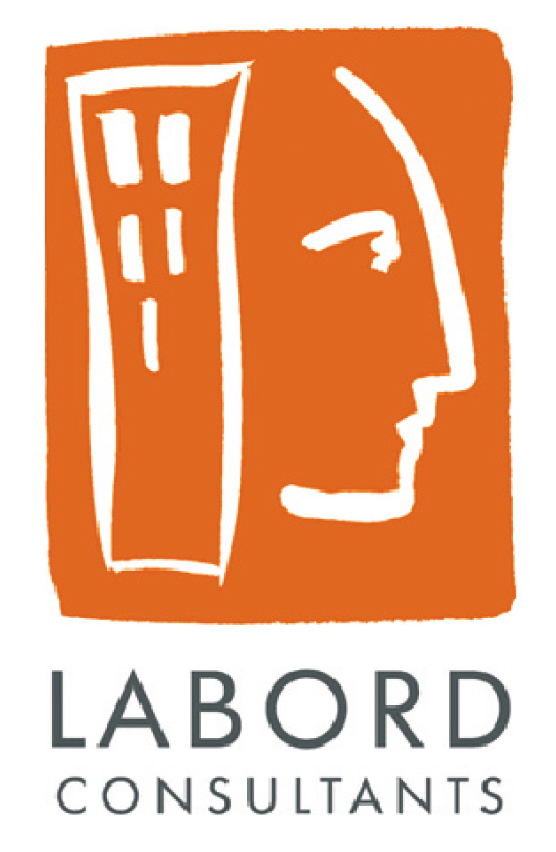The logo image for Labord Consultants features an orange rectangle with painted-like, textured edges taking up the top two-thirds of the design. On the left side of this rectangle, there's a white line drawing that resembles a tower or building with distinct windows on three levels, representing the architectural aspect of the logo. On the right side, there's a white outline of a man's face in side profile, complete with a loosely detailed eye, suggesting a human element tied to the tower, perhaps as a representation of creativity or intellect. This arrangement makes the tower appear like the hair of the face. Below the orange rectangle, filling the bottom one-third of the image, is the company name "Laborde Consultants" written on a white background in black text. The word "Laborde," spelled L-A-B-O-R-D-E, is in the same font as "Consultants" but is larger, thicker, and stretched out to match the length of "Consultants" while standing twice as tall. The overall color scheme consists of orange, white, and black, making the design suitable for various corporate uses such as business cards, brochures, and online platforms.